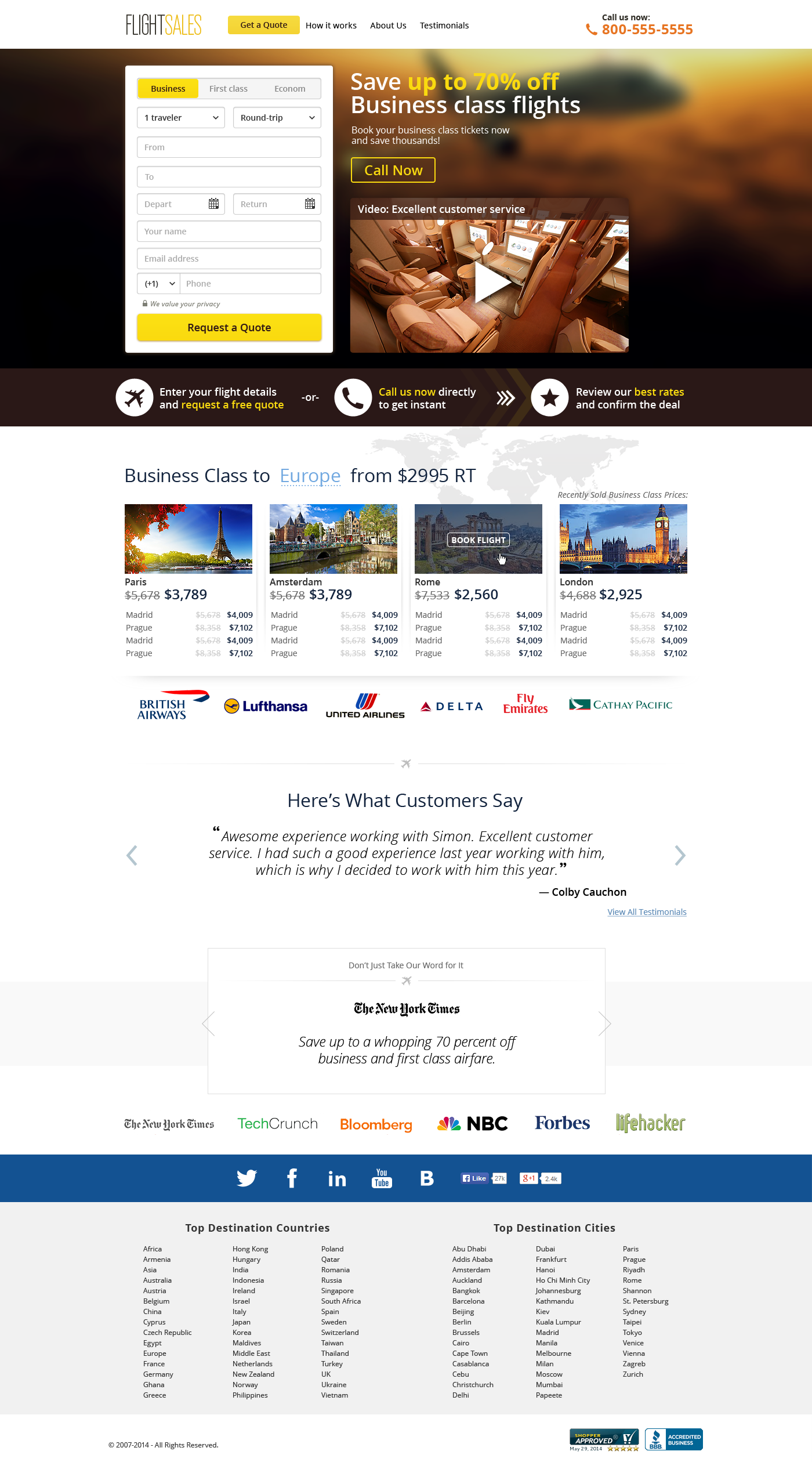This color photograph appears to be a screenshot from a computer or laptop screen displaying an airline reservation website, likely focused on business class flights. At the top of the screen, there's a navigation bar featuring options such as "Flight Sales," "Get a Quote," "How It Works," "About Us," and "Testimonials." On the upper right-hand side, there is a call-to-action section that says "Call Us Now" alongside an icon of a phone receiver and the contact number 800-555-5555.

Below the navigation bar, a prominent rectangular photograph showcases the interior of an airplane's business class section. Overlaid text reads, "Save up to 70% on Business Class Flights." To the left of the photograph, a booking form allows users to select their travel preferences, including class options (Business, First Class, Economy), number of travelers, round-trip or one-way options, departure and destination locations, and departure and return dates. The form also requires personal details such as the traveler's name, email, and phone number, and includes a "Request a Quote" button for submitting the information.

Further down, instructions prompt users to enter their flight details or call directly for an instant quote, emphasizing the availability of immediate assistance and competitive rates. Following this, a section titled "Business Class to Europe" displays four windows with pricing details for various European destinations, offering a transparent view of potential travel costs.

The bottom of the page features customer testimonials, with a bullet point header stating, "Here's What Customers Say," providing a glimpse into previous customers' experiences and satisfaction levels.